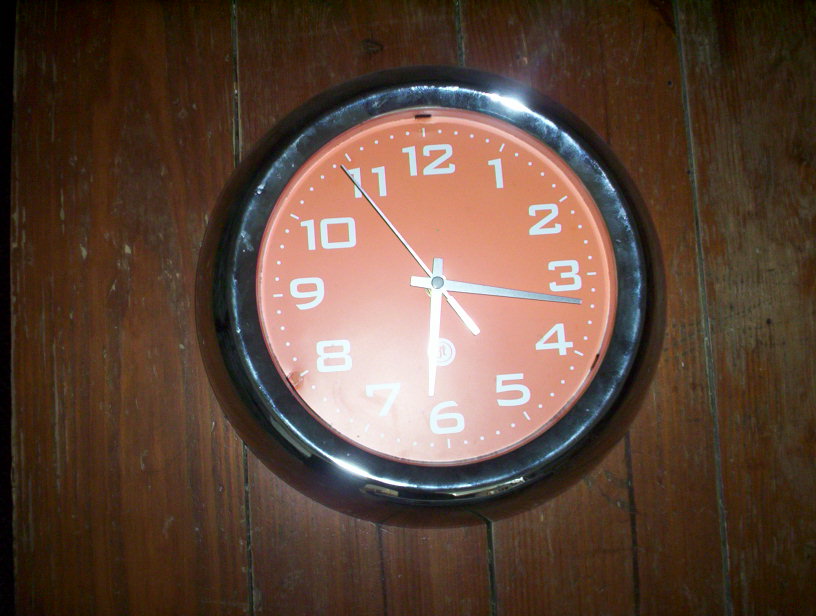This photo features a wall clock with a vibrant orange face and white numerals ranging from 1 to 12. Though the clock's logo is obscured due to focus issues, a noticeable flash reflection suggests the use of a camera flash while capturing the image. The clock's rim appears to be either chrome or a darker material, and it shows signs of wear, indicating it has been mounted for some time. It hangs on an aged, vertically paneled wooden wall, characterized by a dark walnut hue and visible grain, along with signs of wear on the wood, enhancing its rustic appeal.